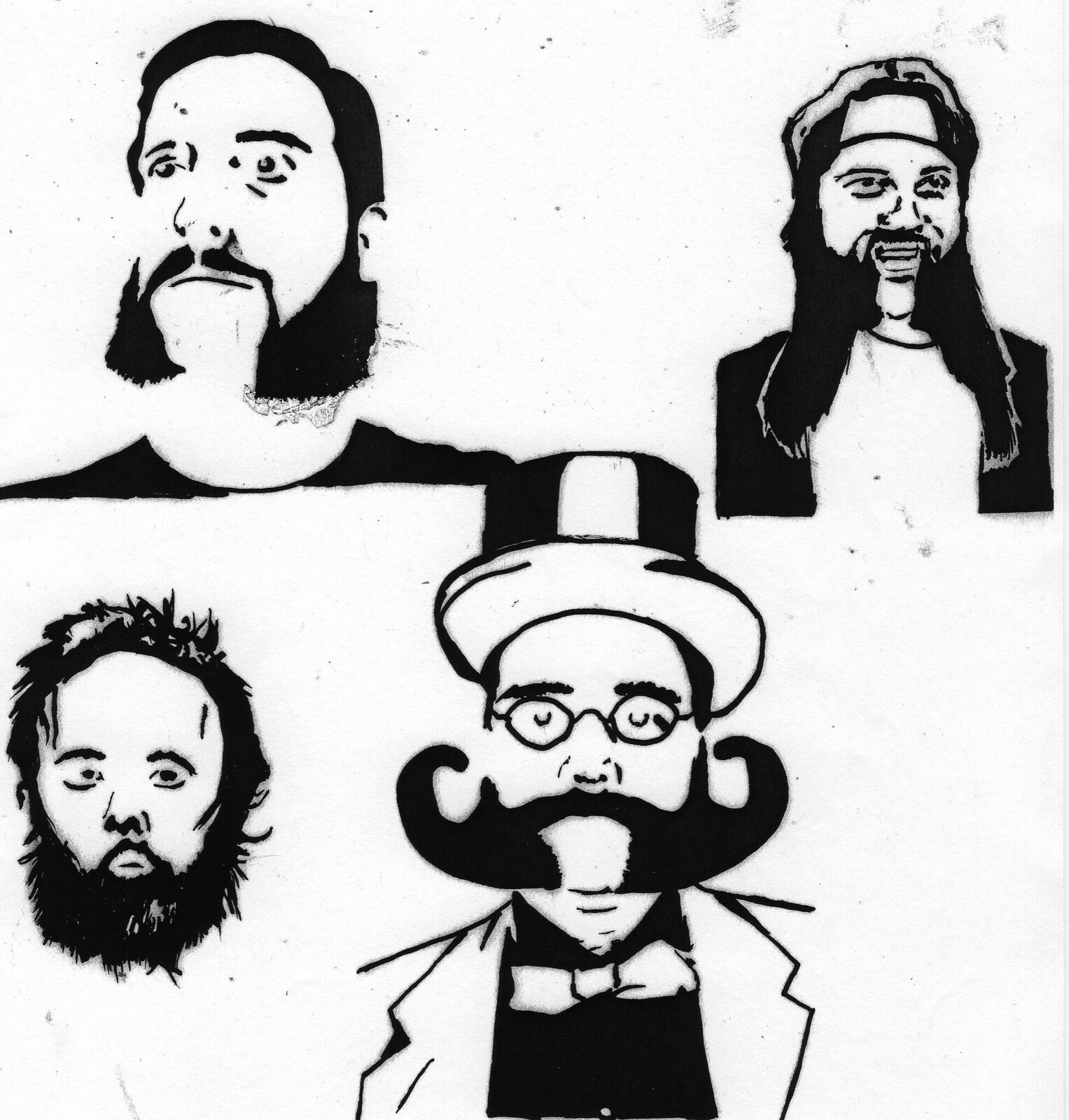The black and white illustration, resembling digital sketch art, showcases a montage of four distinct male portraits, focusing on varied styles of facial hair. The background is predominantly white with black dots and smudges, giving it a textured appearance.

In the bottom left corner, a man with disheveled spiky hair sports a thick, bushy beard that extends well below his chin, complemented by a matching mustache. Adjacent to him in the center bottom, another man dons a vintage look with a large handlebar mustache curling upwards, wearing small round glasses and a top hat. His attire includes a black dress shirt, a white bow tie, and a white jacket outlined in black.

In the top corners, two more men add to the diverse representation. On the left, a man with a mutton-chopped beard, characterized by thin facial hair lines tapering into a fuller beard on the sides, is depicted looking to the left. His hair merges seamlessly with his beard. On the right, a man exudes a hippie vibe with long, shoulder-length hair flowing into his beard. He wears a headband and has a gap in his beard at the chin, with his facial hair forming two flat, ponytail-like strands.

Overall, the image intricately depicts different types of men's facial hair, reflecting a range of styles and eras.